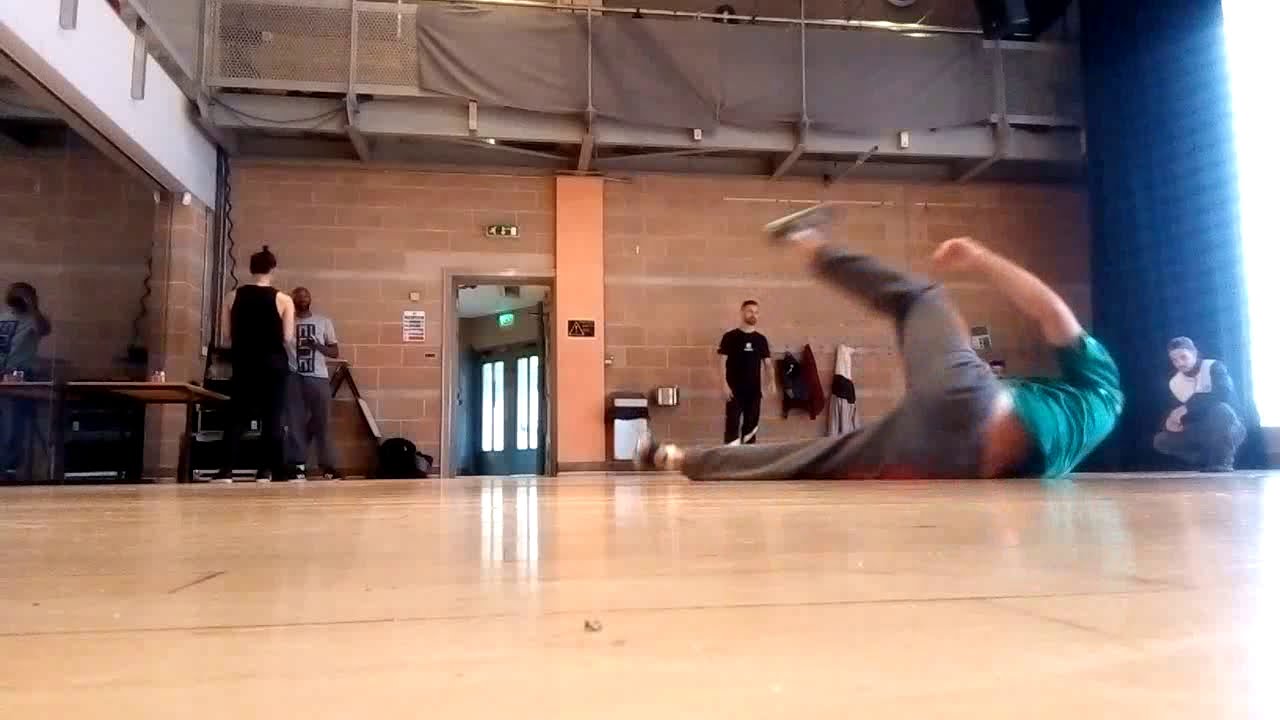This horizontal-rectangular image captures the interior of what appears to be a gymnasium, characterized by a hard, polished wooden floor and a red brick wall extending to the ceiling. In the foreground, a man wearing a green T-shirt and gray or tote pants with sneakers is caught mid-motion, possibly performing a breakdance spin move or falling, with one arm and one leg raised in the air; his blurred limbs hint at dynamic movement. This man is positioned on the floor itself, not a mat, and light reflecting on his skin adds to the visual intensity.

On the left side of the image, two men dressed in black are present: one in a black T-shirt and pants, and the other in a black sleeveless muscle shirt, seemingly engaged in conversation. Mid-frame, towards the right edge, another man is crouched at the base of a blue curtain, appearing to observe the man in the foreground. Behind these figures, a door to the outside with light shining through and an exit sign is visible, adding depth to the scene. Additionally, windows or light leaks on the wall create natural light reflections in the image, enhancing the atmospheric feel of the gymnasium.